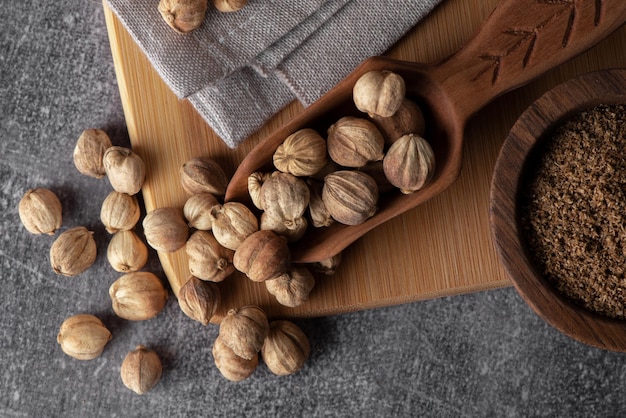The photograph is an overhead shot capturing a rustic arrangement on a table with a gray background. Atop the table lies a wooden cutting board, notable for its warm, contrasting hue. Positioned in the center upper portion of the image is a neatly folded gray napkin. A wooden scoop is strategically placed from the top right, extending vertically towards the bottom left, brimming with whole, unshelled walnuts. These walnuts spill artfully from the scoop onto the cutting board and subsequently, onto the table. In the lower right corner of the wooden board, a small round wooden bowl containing a brown, soil-like substance is visible. The photograph is subtly lit, casting a slight shadow, giving a sense of depth and texture to the nuts, the cutting board, and the other elements within the scene. The arrangement includes approximately 25 walnuts, all with their hard, brown shells intact, and the overall composition exudes a natural, earthy aesthetic.